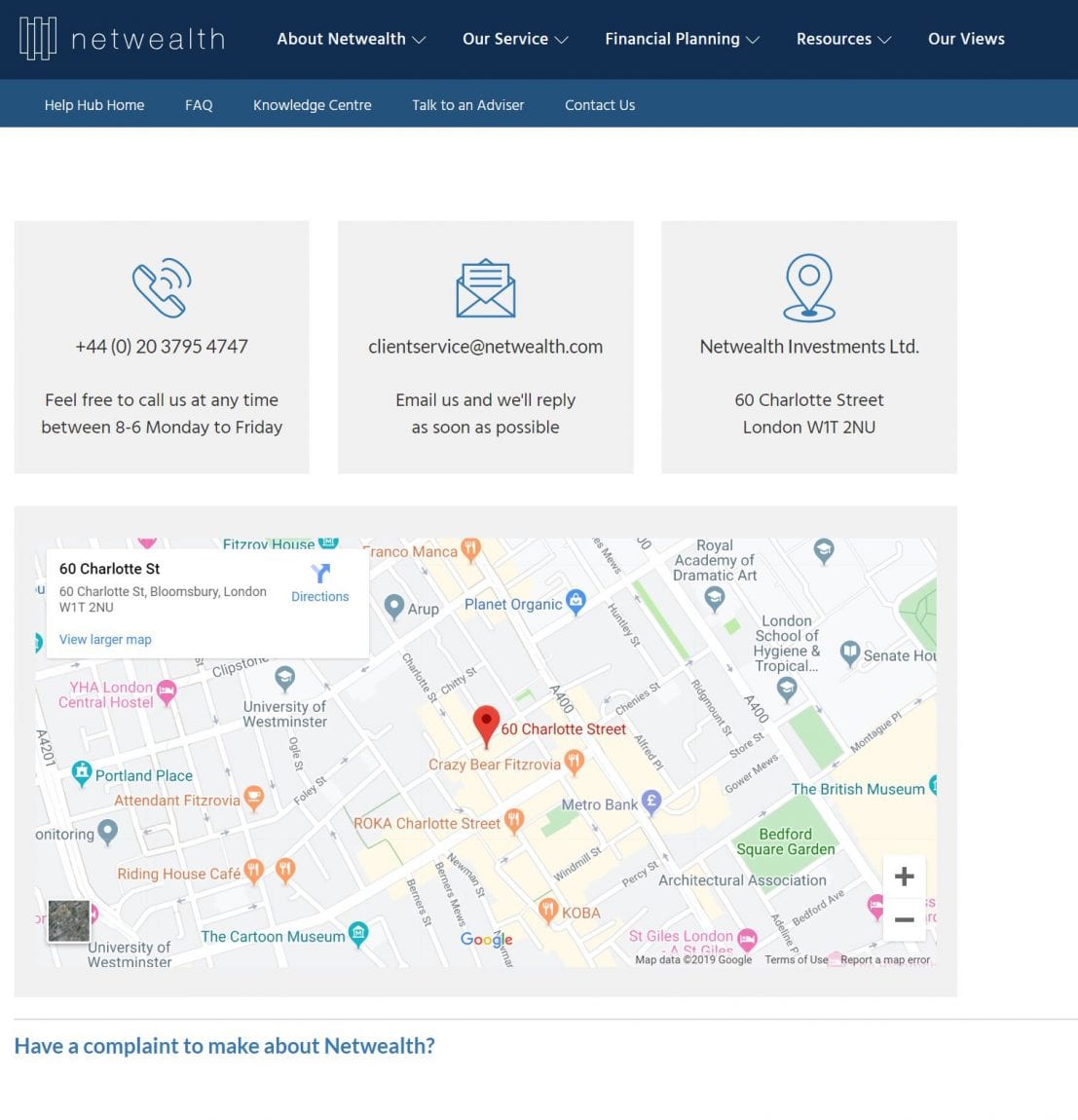This screenshot captures a detailed view of a webpage from the Net Wealth website. At the top, a dark blue banner with white text and down arrows navigates to sections such as "About Net Wealth," "Our Service," "Financial Planning," "Resources," and "Our Views." Below this banner, a lighter blue bar provides further navigation options including "Help Hub Home," "FAQ," "Knowledge Center," "Talk to an Advisor," and "Contact Us."

The central content area features three informative boxes each containing an icon and text. The first box displays a phone icon with a message in gray text, "Feel free to call us at any time between 8 to 6, Monday to Friday," written below a phone number. The second box contains an envelope icon, indicating email communication, with text inviting users to "Email us and we'll reply as soon as possible." The third box features a pinpoint icon, symbolizing a location, with the company name "Net Wealth Investments LTD" and an address beneath it.

The lower section of the screenshot showcases a map, annotated with various markers. Street names are clearly visible alongside different points of interest. Blue shopping bag icons represent shopping areas, a red dot signifies another point of note, and orange bags with forks and spoons indicate restaurant locations.